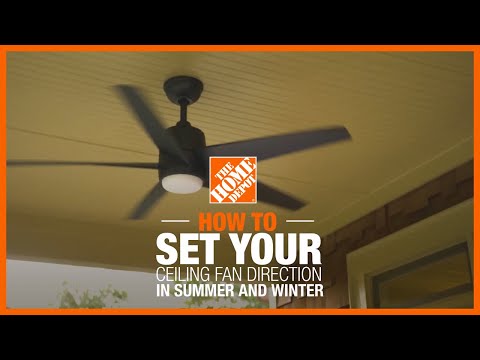This is a horizontal, rectangular ad for The Home Depot. It features black bands at the top and bottom, with an orange outline framing the central image. The picture showcases a dark bronze, five-blade ceiling fan with a cylindrical center and a rounded, white light at the bottom, suggesting it's in motion. The fan is mounted on a yellow ochre paneled ceiling, indicative of an outdoor porch setting, as it includes glimpses of the house’s sideboards, a doorway, and an outdoor window, along with some foliage, hinting at a daylight scene. Dominating the top of the image is The Home Depot logo, accompanied by white dashes. Below it, large block letters read "Set Your," followed by "Ceiling Fan Direction" in smaller letters, and finally, in bold, "In Summer and Winter."